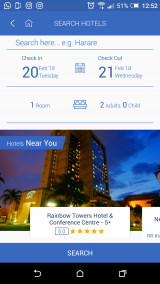This is an intricate vertical rectangular image that serves as a hotel search interface. At the top, there is a blue header with white text reading "Search Hotels," accompanied by a white home icon and a left-facing arrow. Below this header, on a white background, there's a search bar labeled "Search Here," alongside a placeholder example of a location.

Next, there is a section separated by blue lines at the top and bottom, again on a white background with blue text. It displays "Check-In" followed by the potentially black text of "20 February '18, Tuesday." Similarly, the "Check-Out" section shows "21 February '18, Wednesday," with a blue calendar icon situated between these dates.

Following this, another section, distinguished by the same blue lines as dividers, details the room and occupancy information. It reads "One Room" with a blue bed icon beside it, and beneath, it says "Two Adults, Zero Child."

Lower down the image, a colorful photograph of a hotel is displayed under an evening sky with scattered clouds, illuminated by numerous lights, amidst palm trees. A pop-up within the image identifies the hotel as "Rainbow Towers Hotel and Conference Center," rated five stars plus.

Finally, at the bottom, there is a blue search bar overlayed on the white background, followed by a black area hosting three additional icons.